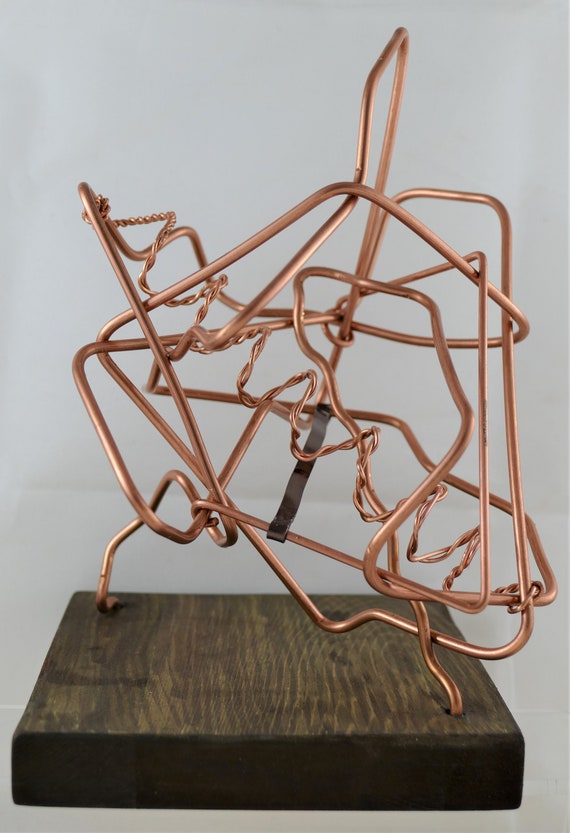This is a color photograph of a three-dimensional metal sculpture mounted on a large square wooden base, which features a slightly faded and lighter wood grain, giving it a yellowish-brown hue. The sculpture predominantly consists of thick, bent copper-colored wires twisted into an abstract, knot-like shape. Interwoven through the larger wires is a thinner, spring-shaped copper wire that forms a spiral, echoing the structure of a DNA helix, and runs diagonally from the top left to the bottom right. Additionally, a darker metal band can be seen attaching two sections of the copper tubing together, though it is unclear if this band is a structural component or part of the artistic design. The sculpture, roughly a foot tall and wide, is presented against a featureless gray or white background, emphasizing the intricate and chaotic yet deliberate arrangement of the copper wires.